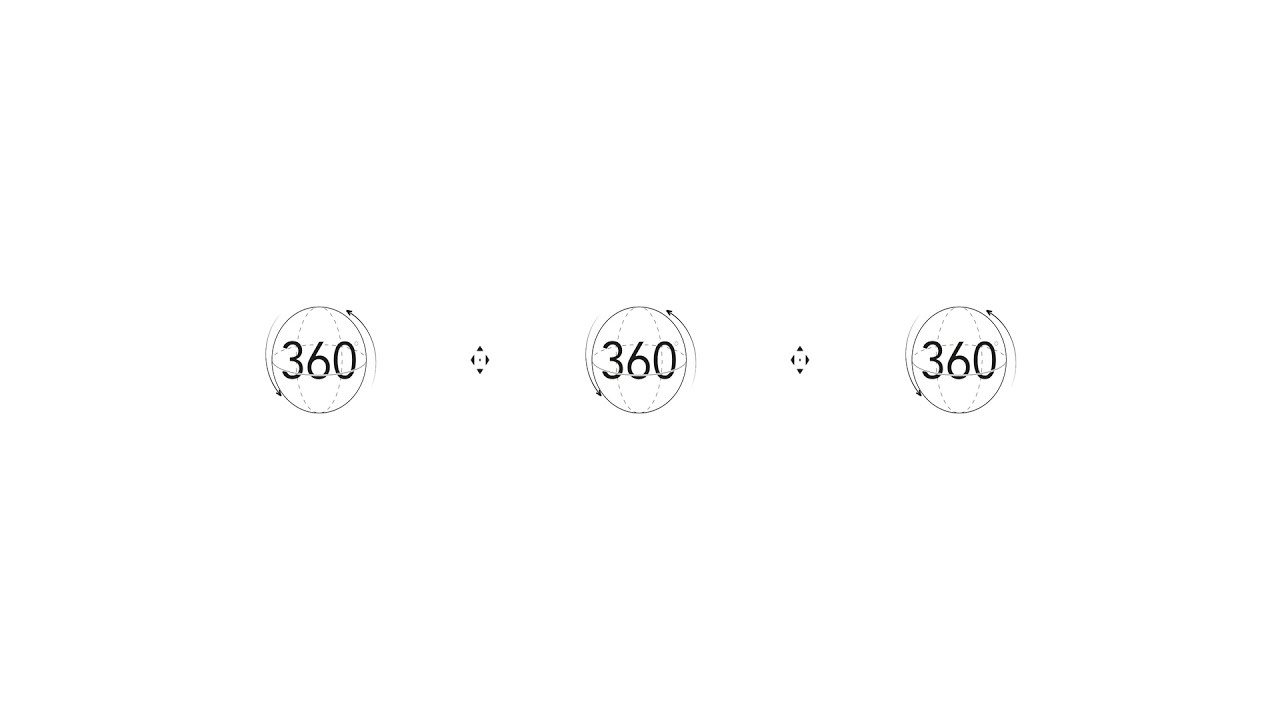This image features three identical black and white globes, each prominently displaying the number "360," arranged horizontally across the center of the white background. These globes have small, curved arrows indicating their rotation—specifically, an arrow on the left pointing downwards and an arrow on the right pointing upwards along the curvature of the globes. In between the globes, there are small multidirectional arrow symbols (triangles) pointing in four directions: north, south, east, and west. The design is minimalistic, focusing solely on the black and white elements, with no additional background or colors.